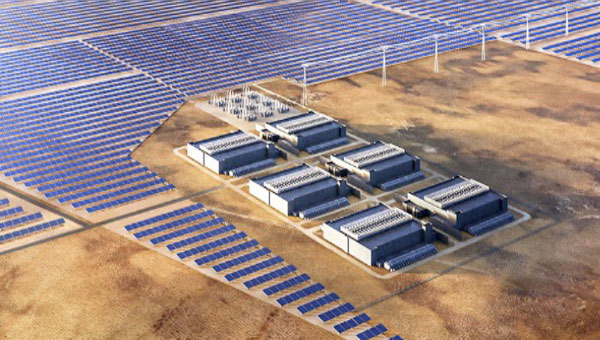This aerial photograph captures a meticulously arranged solar panel farm sprawling across a vast expanse of sandy soil. Thousands of black, glass-like solar panels are meticulously lined up in different shapes, all oriented diagonally from the top left to the bottom right of the image. Nestled in the center of this massive field are six identical one-story buildings, each featuring a blue roof and walls that alternate between blue and a grayish-white hue. These buildings likely serve as energy storage facilities. Adjacent to them, a second field contains nine smaller structures, whose purpose remain unspecified. Additionally, white windmills dot the landscape, contributing to the renewable energy collection. Several light posts and white power lines are also visible, stretching from the middle to the top of the photograph, adding to the intricate infrastructure of this renewable energy facility.